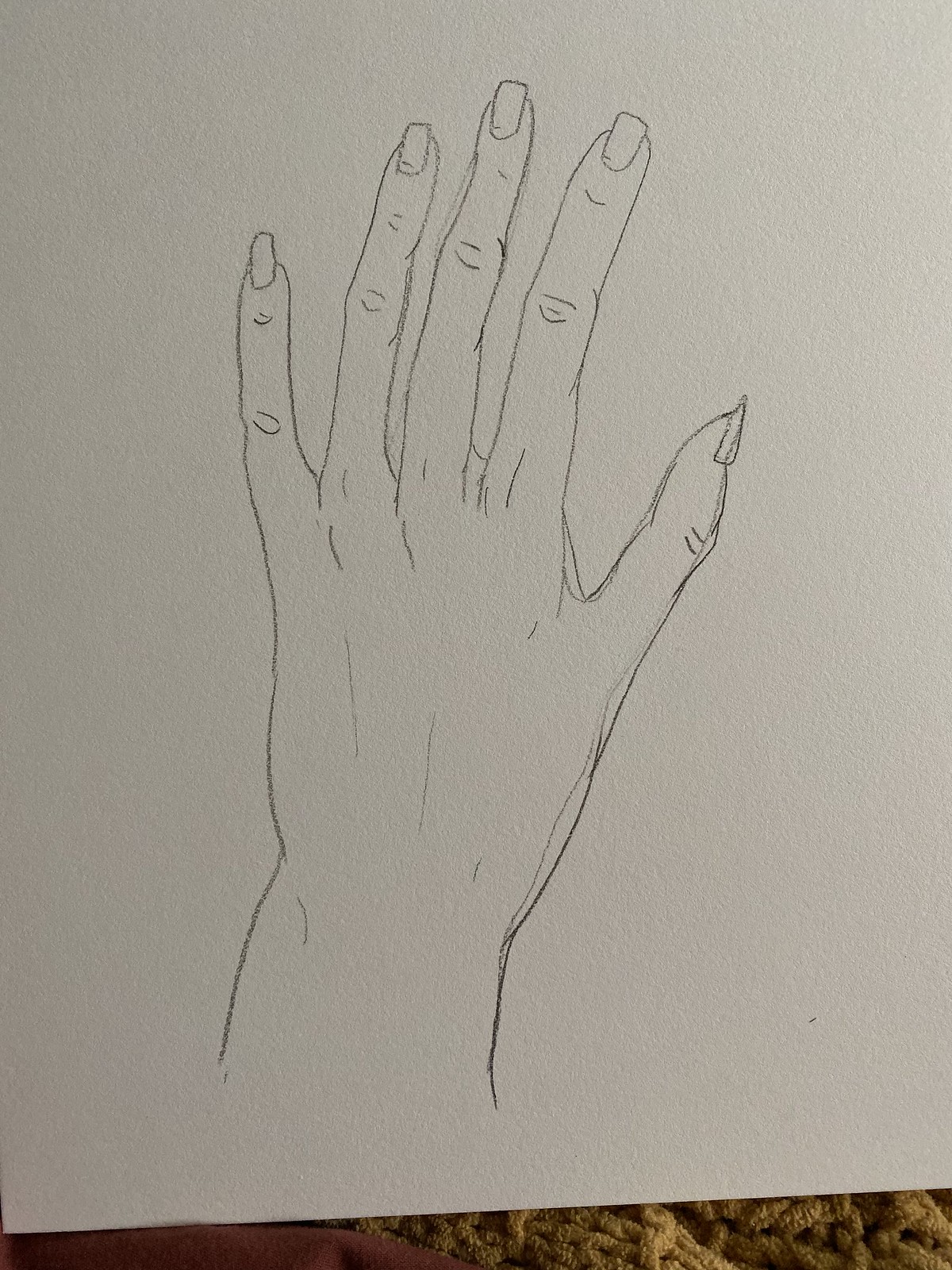The image features a photograph capturing a detailed drawing of a hand. Occupying approximately 90% of the frame, the drawing is rendered on a pristine white piece of paper. The hand depicted is anatomically typical in shape, showcasing a wrist, palm, four fingers, and a thumb. However, the fingernails are unusually elongated and irregularly proportioned, evoking a somewhat eerie quality akin to claws, though not quite as menacing.

In the lower left corner of the image, part of a real hand is visible, providing a stark contrast between the drawn and the actual. Meanwhile, the lower right corner reveals a piece of fabric, possibly a sheet, adding a layer of texture to the composition. The detailed yet unnerving elements of the drawing create an intriguing juxtaposition with the real hand and fabric.